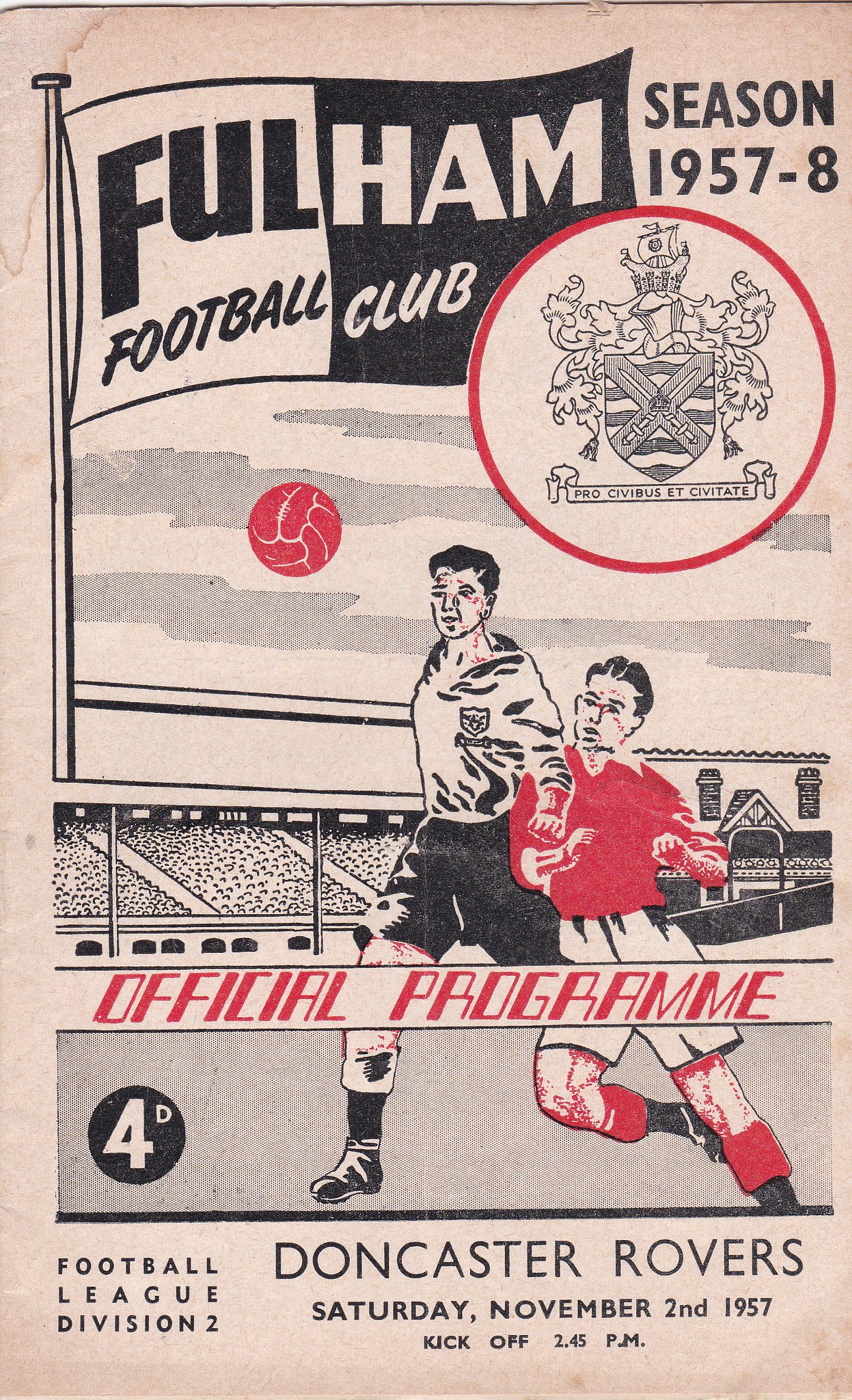The image is the front cover of an old, worn-out official program for a Fulham Football Club match during the 1957-58 season. The paper appears aged and slightly brown. Across the top left, there's a flag that is two-toned, divided into white on one side with black writing, and black on the other with white writing, stating "Fulham Football Club." Adjacent to the flag, the text "Season 1957-8" is positioned, alongside a crest encapsulated in a red circle with the Latin phrase "Pro Civibus et Civitate."

Dominating the bottom right section of the cover, two drawn soccer players are intensely vying for a soccer ball, which is in red and situated slightly above them to the left. One player is dressed in black shorts with a white and black top, while the other wears a red top and white shorts. Both players appear somewhat bloodied, adding a dynamic element to the scene.

In the background, there are stands filled with spectators, emphasizing the setting of a competitive match. The program lists key details in red and black ink; below the players, it reads "Doncaster Rovers, Saturday, November 2, 1957, Kickoff 2.45 p.m." The text "Official Program," "Football League, Division 2," and Fulham Football Club details, including the crest and image, are all prominently featured, culminating in a rich depiction of a historic soccer game.